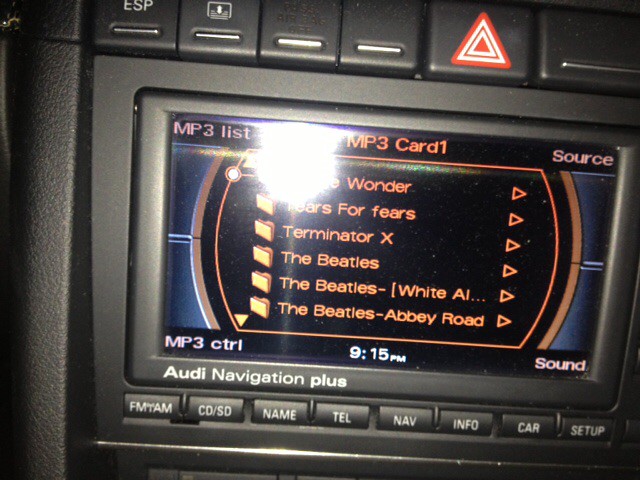This close-up image of an Audi primary console reveals a sleek, black interior with a prominent central navigation screen in music mode. The menu, displayed in orange text, lists MP3 files including tracks from Tears for Fears, Terminator X, and The Beatles with their iconic albums like the White Album and Abbey Road, each accompanied by a small folder icon and outlined play button. The screen also shows a clock reading 9:15 PM and bears the branding "Audi Navigation Plus" at the bottom left. Surrounding the display are several operational buttons such as FM, AM, CD, and SD, with a red and white hazard lights button visible at the top right. The entire setup, reflective of high-tech automotive design, is accentuated by metallic detailing and exhibits features for audio, radio, CD, telephone, and navigation control.